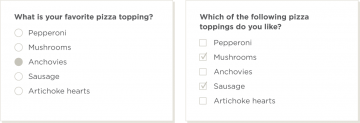This image is a screenshot of an online pizza preferences survey featuring two large square sections, each containing a distinct question in black text. 

The first section poses the question: "What is your favorite pizza topping?" accompanied by five answer options, each with a circular bullet point:
1. Pepperoni
2. Mushroom
3. Anchovies (selected, indicated by a filled gray circle)
4. Sausage
5. Artichoke hearts

The second section asks: "Which of the following pizza toppings do you like?" below which are five choices, each with a square checkbox:
1. Pepperoni
2. Mushrooms (selected, indicated by a checked gray square)
3. Anchovies
4. Sausage (selected, indicated by a checked gray square)
5. Artichokes